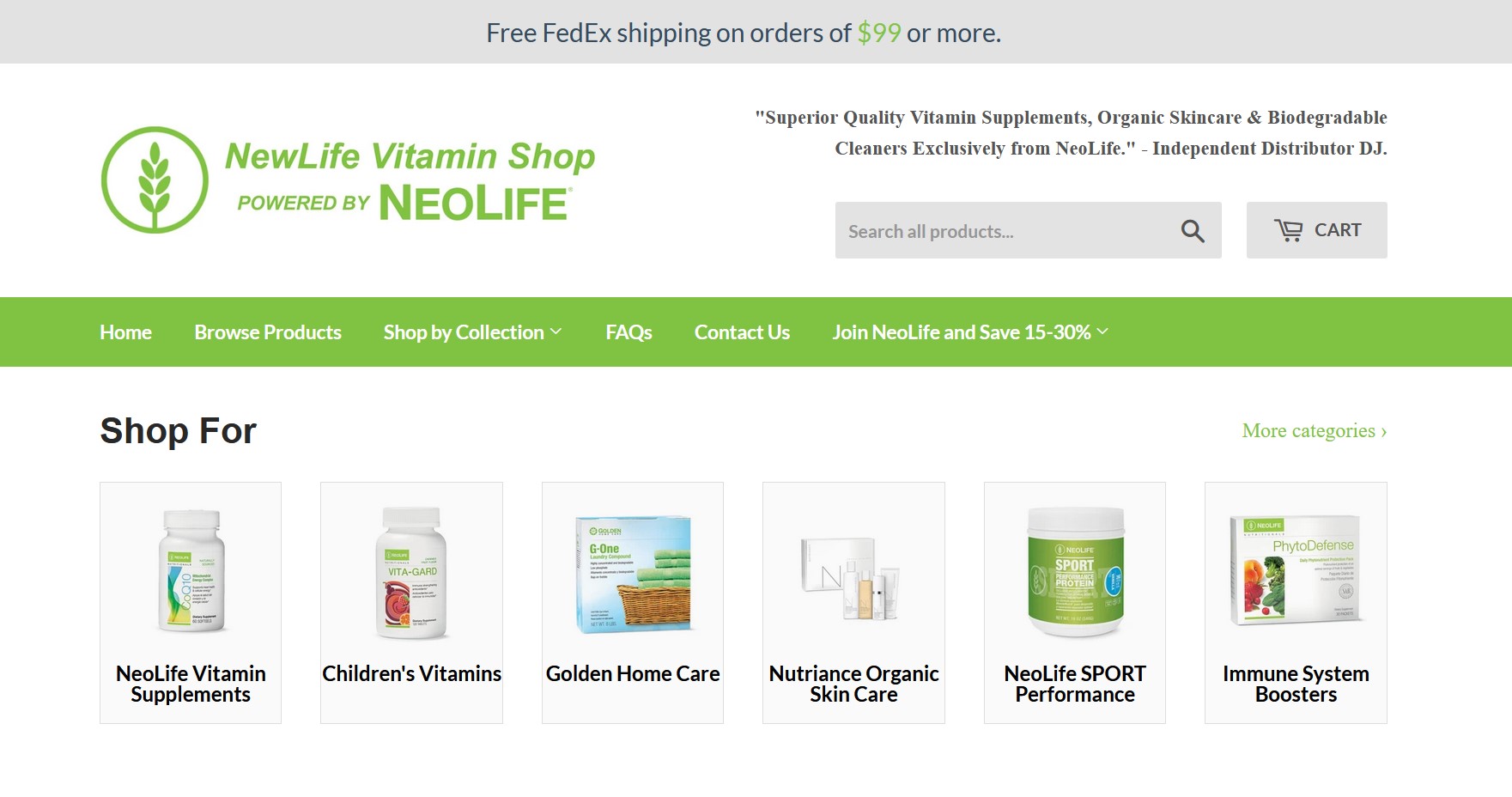The homepage of the website, dedicated to vitamins and health food, is visually appealing with an organized layout set against a clean white background. The header, a gray horizontal bar, features a central message in black font reading, "Free FedEx Shipping on Orders of $99 or More," with the "$99" highlighted in green for emphasis.

Below the header, a white section contains a green outline circle on the left, with a white interior and a green leaf illustration. Adjacent to the circle, the text "New Life Vitamin Shop" and "Powered by Neolife" are displayed in green. To the right, a black font quote states, "Superior quality vitamin supplements, organic skincare, and biodegradable cleaners exclusively from Neolife." The line "Independent Distributor DJ" is included just below.

A gray search box labeled "Search all products" and a gray cart icon follow under this section. Below, a long rectangular green banner provides navigation options in white, including "Home," "Browse Products," "Shop by Collection," "FAQs," "Contact Us," and "Join Neolife and Save 15 to 30%."

The main content area lists product categories such as "Neolife Vitamin Supplements," "Children Vitamins," "Golden Home Care," "Nutrition," "Organs," "Skincare," "Neolife Sport Performance," and "Immune System Boosters," each accompanied by corresponding thumbnails.